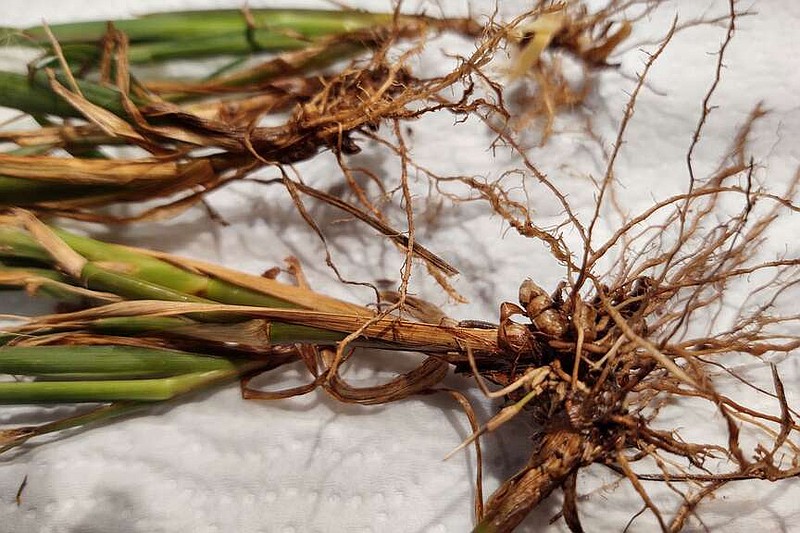The up-close color photograph shows a root vegetable, possibly green onions or scallions, that has been pulled out of the ground and cleaned. The roots are wiry, hairy, and brown, and they lie on a white paper towel, which can be identified by its circular indents resembling those of a Bounty paper towel. The plants' green tips and narrow stems are visible on the left, with some dead, tan-colored outer shells of the stems also present. The roots are neatly arranged horizontally across the paper towel, emphasizing their cleaned, dirt-free state.